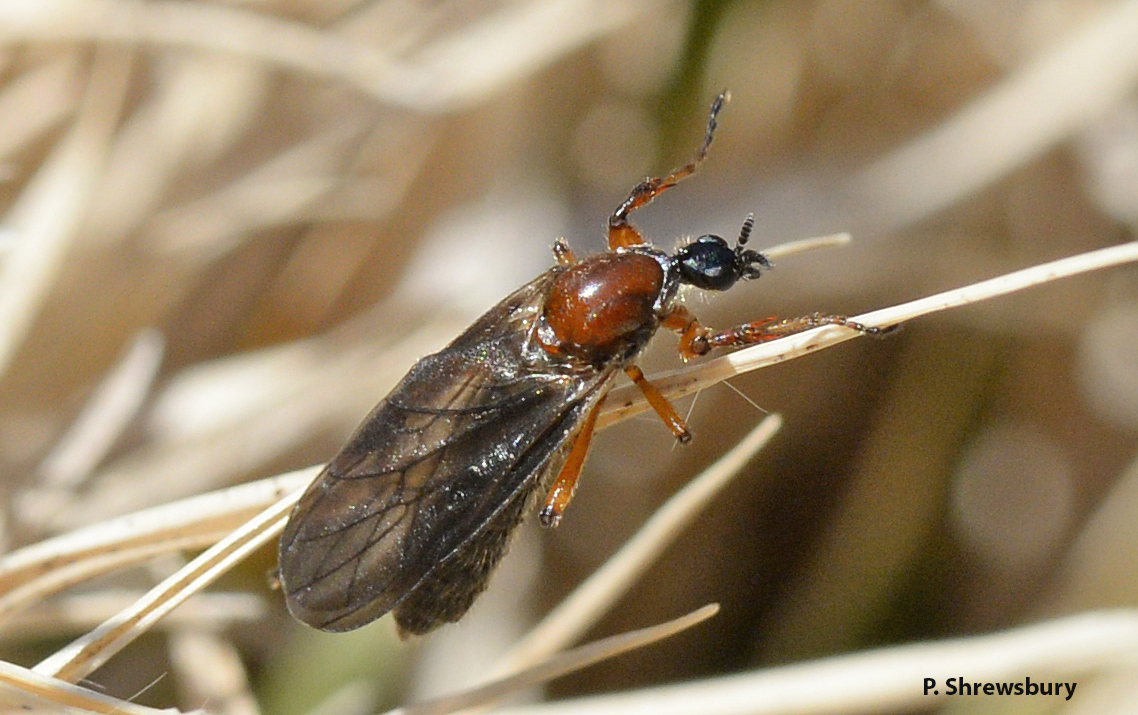This close-up photograph taken by P. Shrewsbury features an intricately detailed insect, possibly a fly, with a prominent position at the center of the image. The fly is perched on a thin, light-colored twig or stem, which stands out in sharp focus against a backdrop of blurred vegetation. The insect's head is black with visible antennae, and its body is predominantly brown with segments of orange and black. The legs, similarly colored, reveal detailed segments, with some extending upwards and others anchoring it to the twig. Dominating the left side of the image, the fly's wings are a mix of black and gray with prominent veins, providing a semi-transparent view through them. The right wing appears darker and more opaque, and hints of another wing can be seen beneath it. The name P. Shrewsbury is inscribed in black font at the bottom of the image, crediting the photographer for this detailed capture.